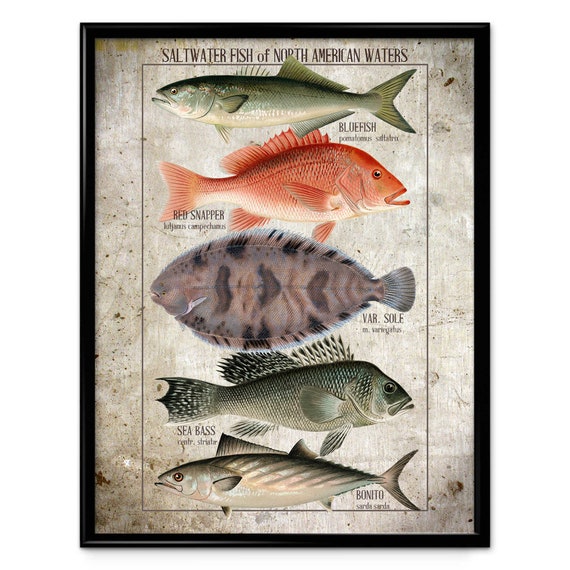The image depicts a detailed, framed poster titled "Saltwater Fish of North American Waters." The poster features a vertical arrangement of five illustrated fish species, each uniquely labeled and detailed. The fish are stacked in alternating directions and are framed within a thin black border. The background of the poster is a weathered, dirty white with brown and black spots.

At the top, the silver and greenish-blue Bluefish is depicted. It has a sleek, torpedo-like body with a white underbelly, black eyes, and open mouth. Following is the Red Snapper, which is a vibrant orange-red with a rounded, oval body and a white underbelly. Its eyes are black, and its mouth is open. In the middle of the poster, there is the Nabs Sole, resembling a flounder, with an oval-shaped body, tiny tail fin, and gray with a striped pattern. It has fins running along the top and bottom perimeters of its body. Below this, the Sea Bass is shown, characterized by its slender, torpedo-shaped body, a little hump behind its eyes, greenish-gray scales, and spiked dorsal fins. Finally, at the bottom, the Bonito fish appears sleek and muscular, similar to a tuna, with dark green to gray scales and hints of yellow or gold, making it appear shiny.

This detailed and visually engaging poster not only names the fish but provides a clear representation of their unique features, all encompassed within a striking black frame.